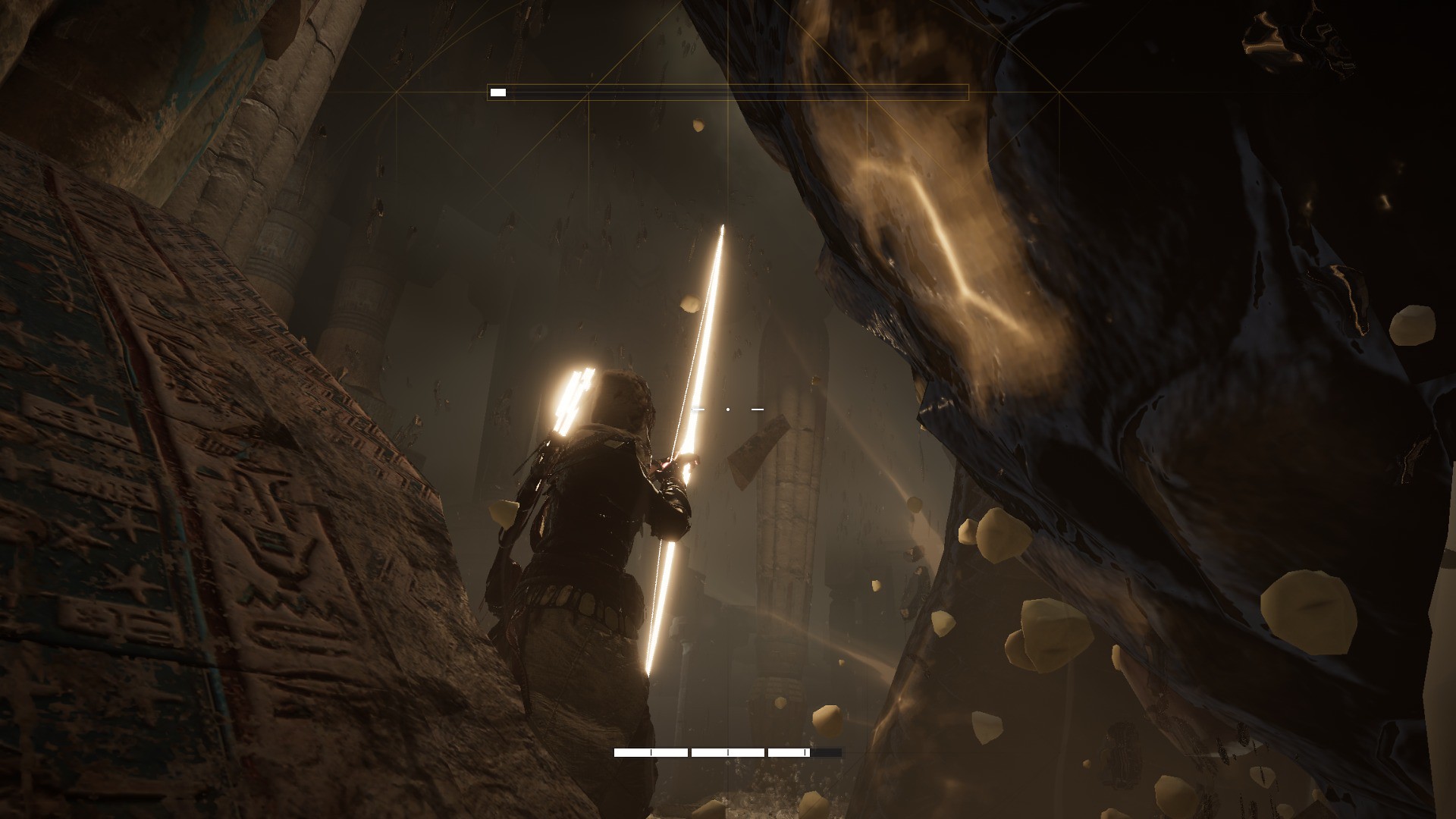In the screenshot of a gameplay scene, a progress bar with a gold outline and a small amount of white fill is prominently displayed at the top of the image. Below it, a humanoid figure clad in a military-style tactical outfit stands poised. The character is adorned with a thick black vest that features a white protrusion emerging from its back and is outfitted in thick cargo pants. The figure is armed with a white saber, though their facial features remain indistinct. Surrounding the character are tan and black stone ruins inscribed with hieroglyphics, suggesting an ancient or mystical setting. The background reveals a dark sky from which rock-like objects appear to be falling. Columns in tan and brown hues are visible, adding to the decrepit ambiance of the ruins. In the foreground, a partially glowing rock structure emits a faint yellow light. At the bottom of the image, another white progress bar is displayed, likely indicating game status or player health.